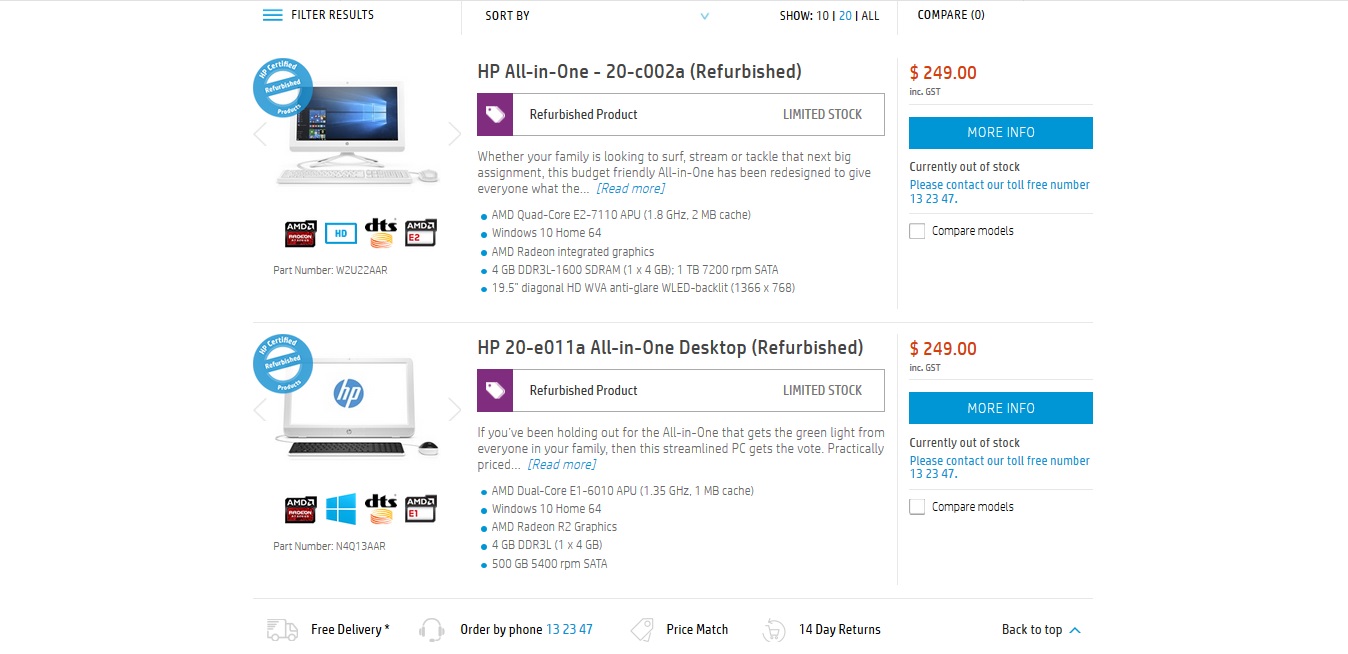The image showcases a website dedicated to the sale of computing products, featuring a search result for refurbished HP desktop all-in-one systems. Both units are listed at a price of $249 each. It appears that the user conducted a search within a specific price range, focusing on computers available for up to $249. Though it’s not clear if this is an official HP site, both displayed products are HP desktop-style computers.

Detailed descriptions accompanying the products include specifications such as the operating system (Windows 10), memory (4GB), screen sizes, and hard drive capacities. Additionally, small icons indicate that the systems come with a keyboard and mouse, and highlight common features like DTS audio technology. Both computers are equipped with AMD processors.

For those seeking more information, there is a blue button labeled "More Info" adjacent to each product listing. However, it's noted that the items are currently out of stock, as indicated on the website, but $249 was their previous selling price.